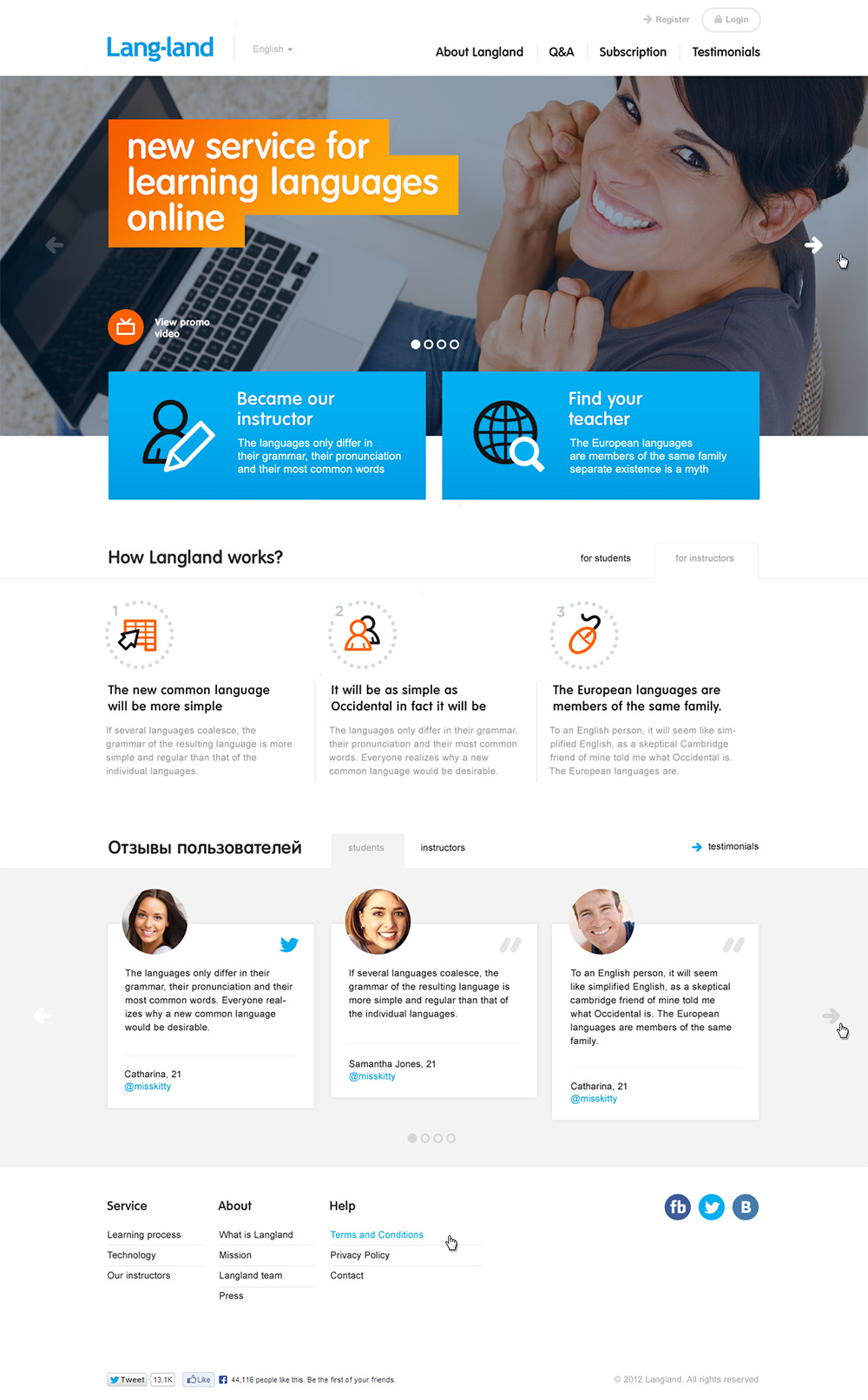This is a detailed vertical image from a website accessible via computer or smart device. The background merges seamlessly with the white of a computer screen, lacking any defined border.

At the top left, the website's logo "Langland" is displayed in blue, accompanied by a language selection option set to "English." Opposite this, in bold black font, are navigation links: "About Langland," "Q&A," "Subscription," and "Testimonials." Above these links, in a lighter grey font, are buttons for "Register" and "Login."

Below the navigation menu, there is an image of a cheerful woman sitting at a desk with a laptop. Her hands are clenched into excited fists near her face as she smiles and looks upward towards the camera. Overlaying this image, an orange banner announces, "New service for learning languages online." Below this, the page indicates that more pictures can be accessed by scrolling.

Prominent call-to-action buttons are included: an orange button labeled "View Promo Video," and two blue buttons marked "Become Our Instructor" and "Find Your Teacher." Additionally, there are selectable options detailing "How Langland Works for Students" and "How Langland Works for Instructors."

Further down, the text discusses the simplicity and commonality of the "New Common Language," comparing it to Occidental languages and mentioning that European languages belong to the same family.

The page contains phrases in various languages and provides separate sections for "Students" and "Instructors." The "Testimonials" section features user feedback and information about different people. Finally, the bottom of the page has links to "Services," "About," "Help," and other clickable options.